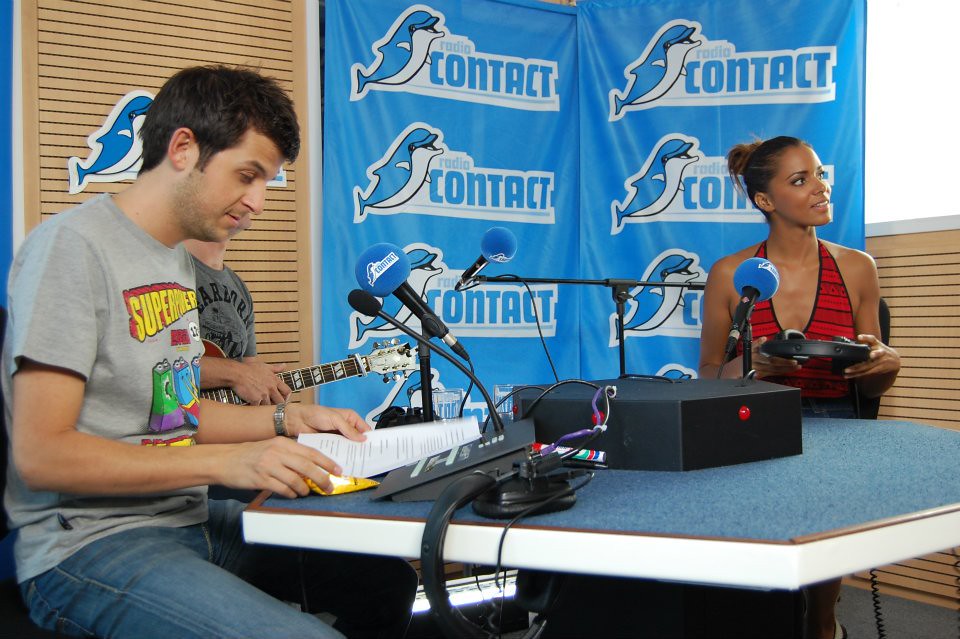The photo features a radio booth scene with three individuals gathered around a table. On the right side, a woman with her hair up and dressed in a red tank top holds a headset while looking away and talking to someone. In front of her, a man in a superhero t-shirt and jeans is intently reading from a script. Both of them are seated in front of blue banners adorned with a dolphin logo and the word "Radio Contact" stacked on top of each other. A third gentleman, partially obscured, is seen in the background holding a guitar. The table in front of them is equipped with several microphones, each covered with large blue foam windshields emblazoned with the radio station's logo.